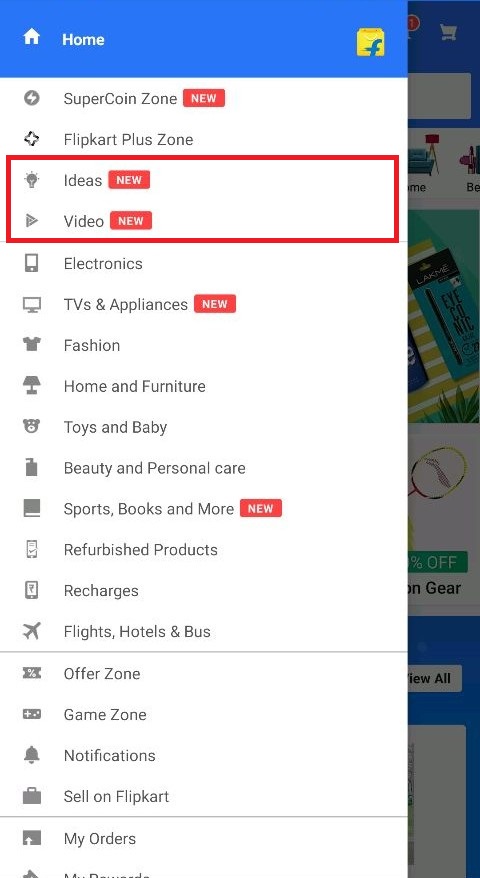The image depicts a predominantly white and blue themed interface, most likely from the Flipkart website or mobile application. A large menu window occupies about 75% of the screen, obscuring much of the background content. At the top of this menu, a blue navigation bar features a "Home" button and a yellow Flipkart logo with a lowercase "f" on the right side.

Below the blue bar, various sections are listed, each clickable for easy navigation. The sections include "Super Coin Zone" with a "New" label next to it, "Flipkart Plus Zone," and "Ideas New" along with "Video New," both of which are highlighted with a red rectangle for emphasis. Other accessible categories include "Electronics," "TV & Appliances," "Fashion," "Home & Furniture," "Toys & Baby," "Beauty & Personal Care," "Sports," "Books & More," "Refurbished Products," and "Recharges." Additionally, there are sections for "Flights & Hotels & Buses," "Offer Zone," "Game Zone," "Notification," "Salon Flipkart," and "My Orders."

Though partially obscured by the menu, the background offers a glimpse of the main website or application interface. Visible elements include text, various items like a couch, and what appears to be a piece of cloth, indicating a storefront or product browsing environment. The cohesive blue and white color theme suggests a clean, modern design consistent with e-commerce aesthetics.